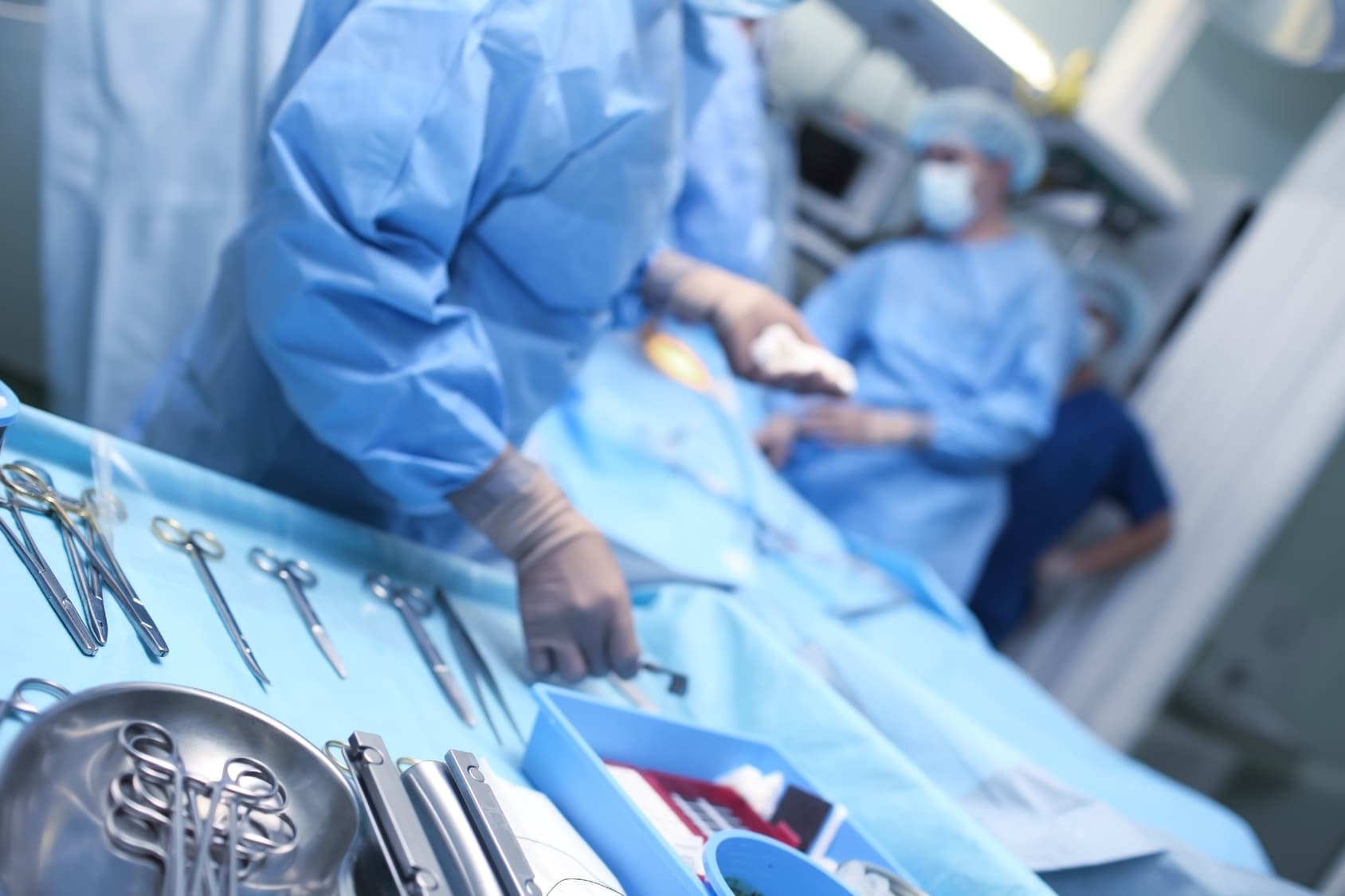This photograph captures a bustling operating room where a surgery is about to be performed. The scene is set with a predominant light blue color, as nearly everything is covered in light blue cloth, including a sheet that drapes over an assumed patient, not directly visible. The medical staff, dressed in darker blue scrubs, are blurred into the background, while the person closest to the viewer, seen from chest to arms, wears dark gray gloves and is in the midst of picking up a surgical instrument. Though slightly blurry, the instrument appears metallic, possibly a scalpel or another surgical tool. In the other hand, this person holds a white cloth. 

A nearby tray lined with a light blue cover showcases an array of meticulously arranged, bright chrome-colored surgical instruments. These include various types of scissors—both pointed and rounded tips—along with long tweezers. Below the instruments, a metal pan contains additional scissors, and a blue tray with indistinguishable objects resides at the edges of visibility. The image is taken at a slight angle, creating a diagonal composition, which adds a sense of dynamic urgency to the setting. Additionally, there are hints of other colors such as white, yellow, silver, red, and black, scattered within the predominantly blue and silver environment, enhancing the sterile, focused atmosphere of the surgical room.